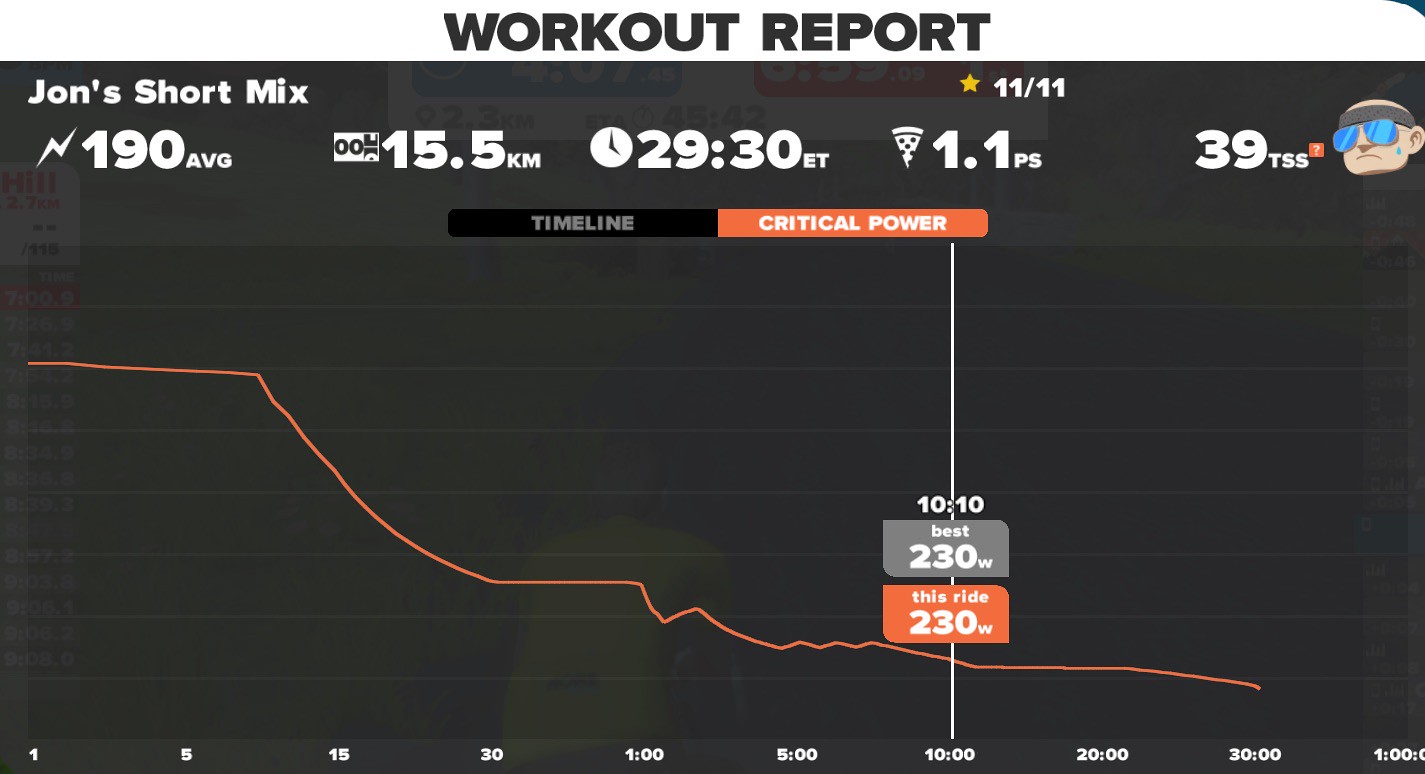This detailed and comprehensive caption describes a screenshot from an app called "Workout Report." At the top of the image, bold black text on a white background clearly states "WORKOUT REPORT." Below this header is the title "John's Short Mix," accompanied by a yellow five-point star with "11/11" beneath the "R" in "REPORT." 

A black graph dominates the center of the image, illustrating various metrics of John's workout. A lightning symbol is positioned below "John's Short Mix," indicating that the average heart rate is 190 bpm. To the right of this, the number "00" is displayed with another partially obscured number. Next to it are statistics indicating a total distance of 15.5 kilometers and a white clock icon with black hands that reads "29:30 ET."

Further details include a slice of pizza icon with "1.1 PS" beside it, suggesting calorie burn or energy consumption. Adjacent to this, the notation "39 TSS" (Training Stress Score) is present with a small red question mark and an illustration of a bald man wearing a black headband and blue sunglasses.

Beneath the clock icon, the graph itself splits into sections labeled "Timeline" on the left and "Critical Power" in white text on an orange background on the right. The x-axis spans from 1 second to 1 hour, marking intervals at 1s, 5s, 15s, 30s, 1min, 5min, 10min, 20min, 30min, and 1 hour. The y-axis indicates power in watts, with highlights showing "10:10" in black and "Best: 230 W" in a gray box. Similarly, " This Ride: 230 W" is marked in orange text. The power graph displays an initial decline with minor spikes, followed by a descent over time.

Overall, the screenshot meticulously documents John's workout details, graphical data on power output over time, and additional metrics contributing to a thorough analysis of the session.